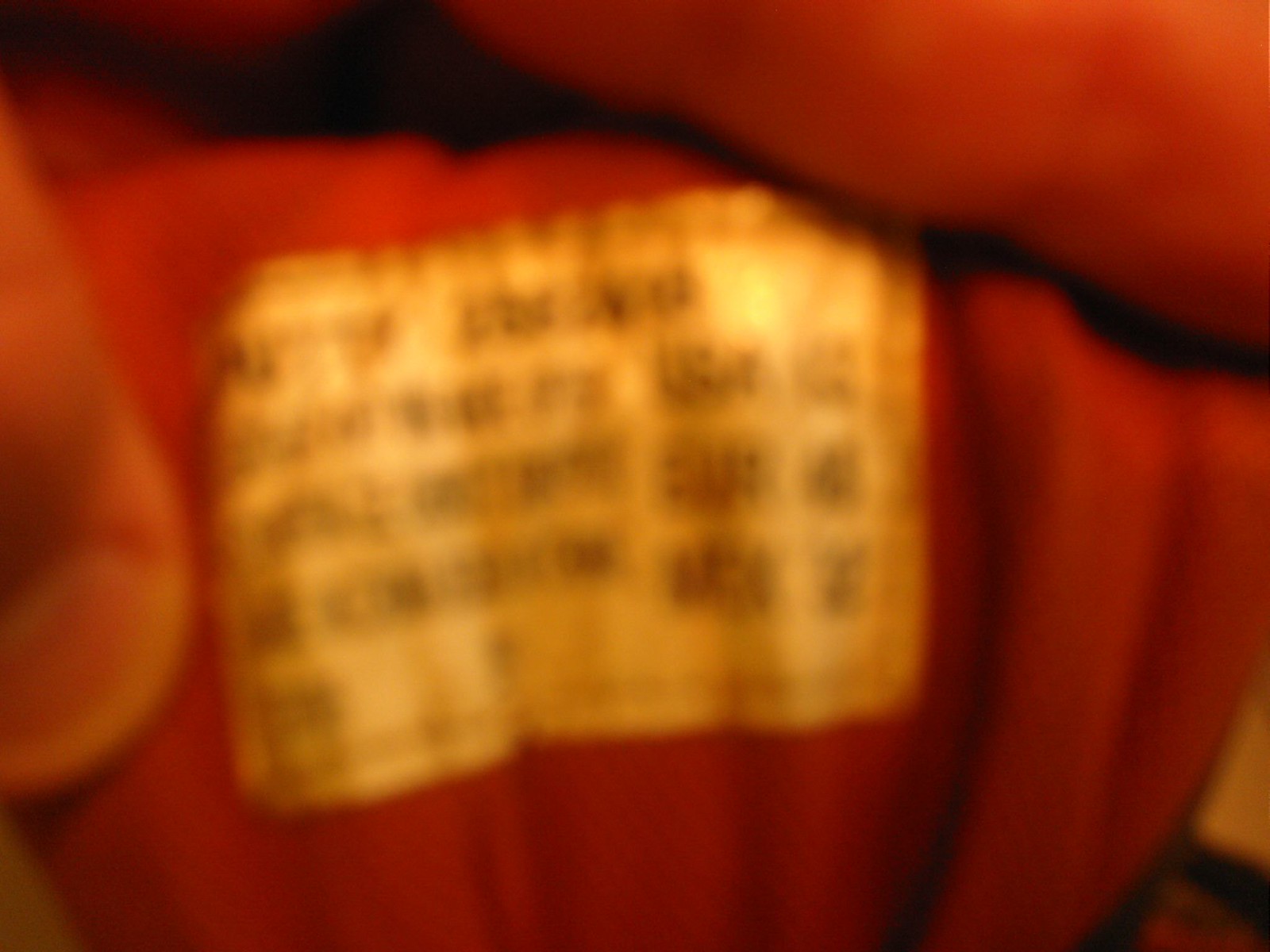This photograph is extremely blurry, capturing a close-up of what appears to be the inside tongue of a red shoe. The image is so out of focus that it's challenging to discern the details. A white label, stitched onto the tongue with red thread, contains several rows of black text that includes size information for different regions, such as the USA and Europe. The text and sizes are nearly impossible to read due to the blurriness. The left side of the image shows a thumb, and the top right reveals a finger, both holding the tongue in place to display the label. The red cloth of the shoe and the manner in which the tag is being held suggest an attempt to document the sizing details, albeit unsuccessfully due to the camera's inability to focus at such a close range.